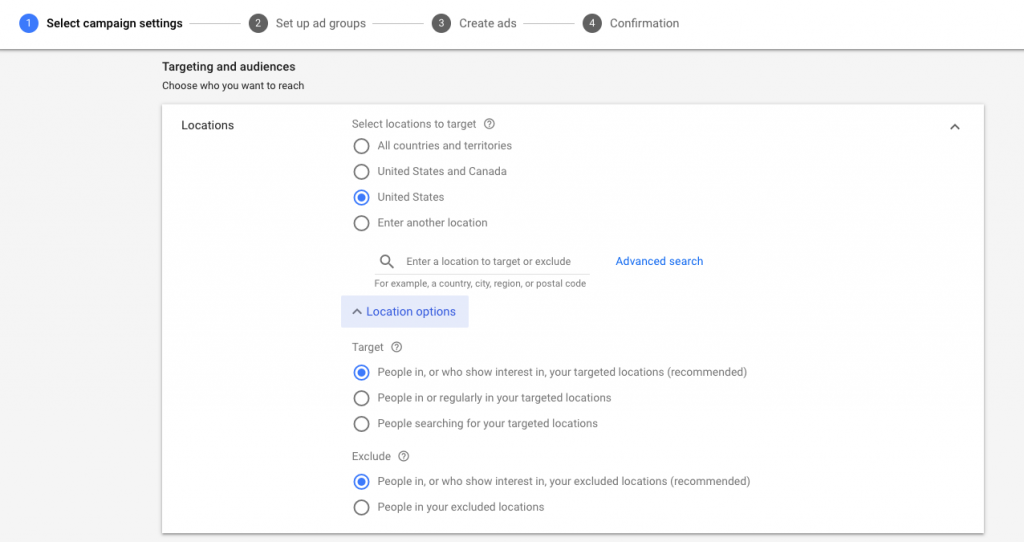This screenshot depicts the campaign settings interface of an online advertising platform, likely used for setting up a political or any other type of promotional campaign. The interface is organized into four sequential steps, displayed horizontally at the top of the screen: 

1. "Select Campaign Settings" (highlighted in blue)
2. "Set Up Ad Groups"
3. "Create Ads"
4. "Confirmation"

Just below these steps, there's a section titled "Target and Audiences," which guides users on choosing their preferred audience reach. In this section, there's a white box labeled "Locations," offering several targeting options:

- "All countries and territories"
- "United States and Canada"
- "United States" (currently selected)
- "Enter another location" (with a text box for input)

Further down, there's a "Target" setting with three selectable options for audience targeting:

1. "People in, or who show interest in, your target locations (Recommended)"
2. "People in, or regularly in, your target locations"
3. "People searching for your target locations"

The first option, "People in, or who show interest in, your target locations," is currently selected.

Lastly, there is an "Exclude" setting to filter out certain audiences, with two available options:

1. "People in, or who show interest in, your excluded locations (Recommended)"
2. "People in your excluded locations"

Here, the first option, "People in, or who show interest in, your excluded locations," is selected.

This comprehensive setup allows users to precisely define their campaign's geographical and audience-specific reach.